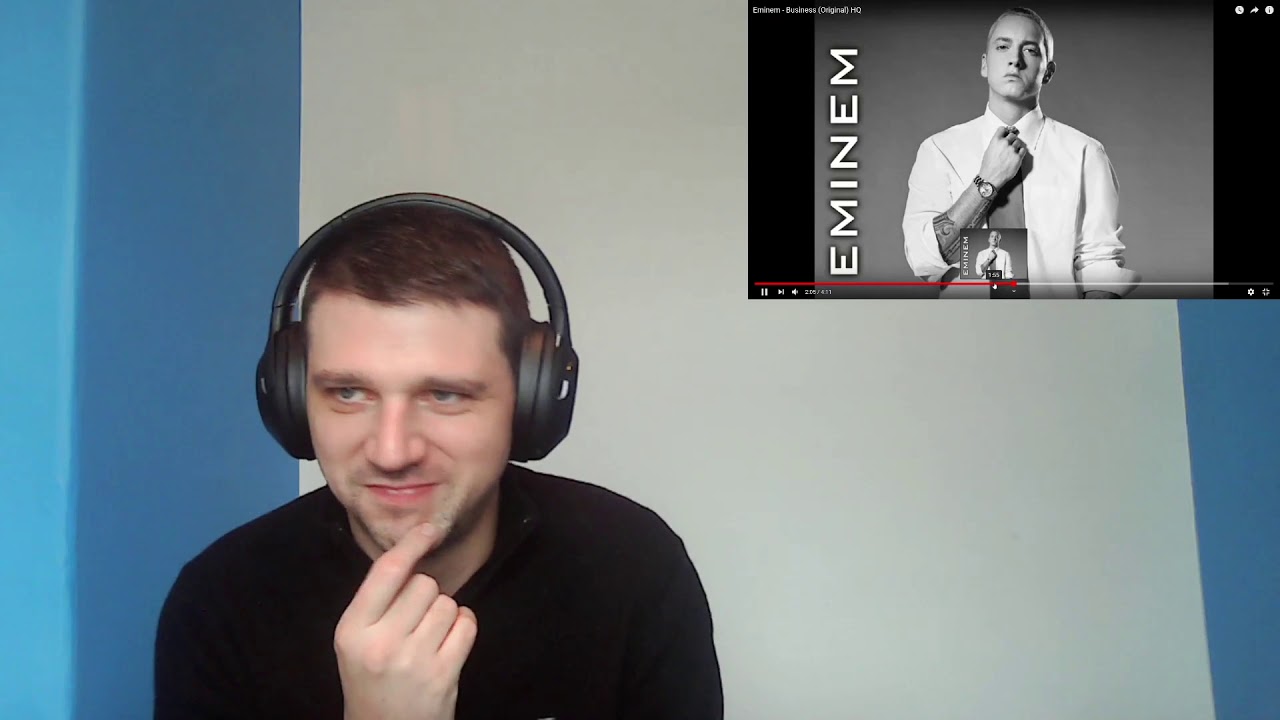In this screenshot from a YouTube vlog, the vlogger is positioned towards the left side of the frame. He is sporting a black headset and has short brown hair. Dressed in a black t-shirt, he rests his hand on his chin, with his index finger placed on the right side of his chin and the rest of his fingers curled into his palm. The vlogger has a thoughtful expression, accentuated by a slight grin, as he looks to the left. His posture is slightly hunched over, and he is seated in front of a wall that is predominantly white with blue sections on either side.

In the top-right corner of the screenshot, an embedded YouTube playback screen is visible, indicating that he is listening to Eminem. The screen features a photo of Eminem with the artist's name displayed vertically along the right side. The iconic red play bar at the bottom of the screen is discernible, along with the pause and volume control icons in the bottom left, and the maximize view icons in the bottom right.